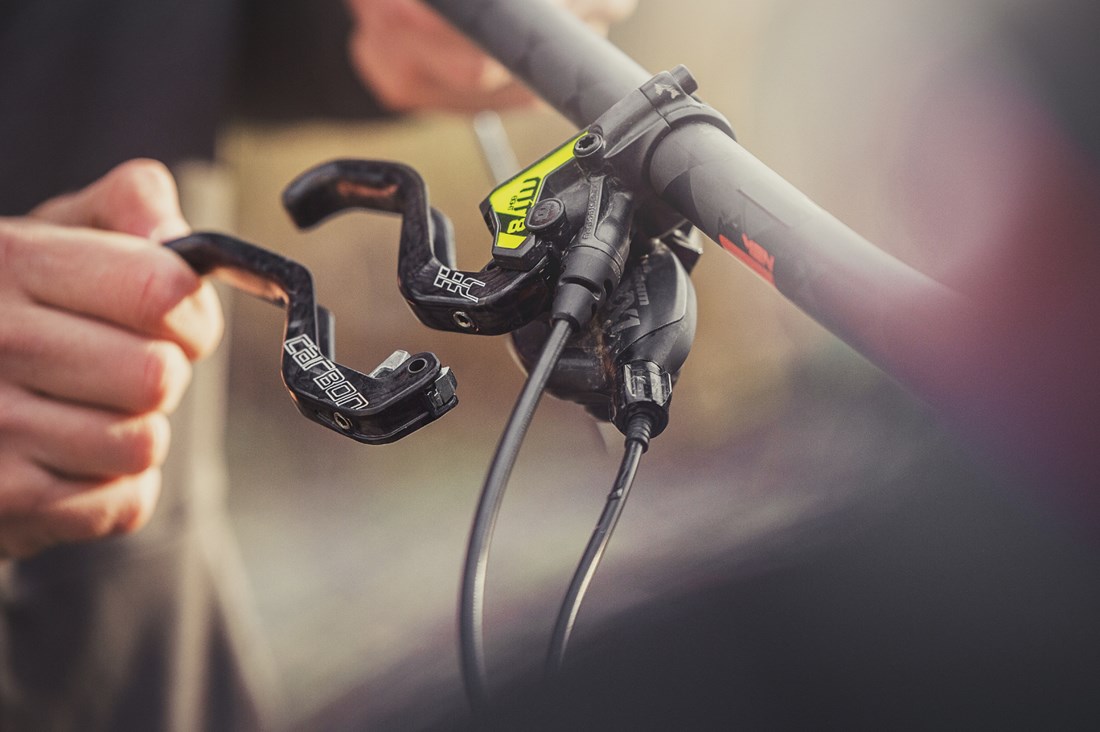The image presents a close-up view of a motorbike handle, specifically focusing on the left handle trigger. The scene is slightly out of focus, showing just the hands, a section of the torso, and the top of the leg of a white male. He seems to be replacing an old handle with a new one. The old handle features the label "HC" while the new one is branded "Carbon." Both handles are predominantly black, with white font logos; the new handle has an additional yellow logo that reads "MT8" above it, though not attached to the handle itself. The man's left hand is gripping the old handle, which has a shifter mechanism—a metal part that needs to be squeezed to shift gears. The setup includes two screws on the handle and some wires, indicating a typical bike handle assembly and replacement process. The old handle appears to be broken, necessitating the replacement.